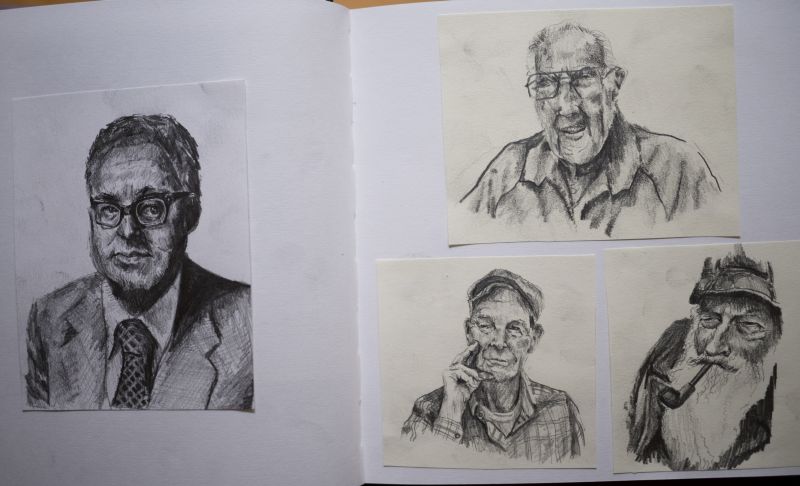The image showcases a collection of four charcoal drawings of men, each adhered to a larger white paper background, which is folded in half and situated on a brown table. The left-hand side features a drawing of a man depicted from the shoulders up, sporting squarish glasses, a suit, a white shirt, and a tie with diamond patterns. The white paper background also reveals subtle charcoal smudges.

On the right, there are three more drawings attached to yellowed pieces of paper. The topmost right drawing portrays an older gentleman with short, spiky white hair, wearing a button-down shirt and glasses. Beneath this drawing, to the left, is a sketch of another elderly man, characterized by a checkered shirt and a hat, with his hand raised to his face. Lastly, on the lower right, there is a depiction of a man with a long white beard, hat, and a long pipe.

Each drawing captures the head and shoulders of the subjects, meticulously detailed in their facial features and accessories, lending a realistic and expressive touch to the overall composition.